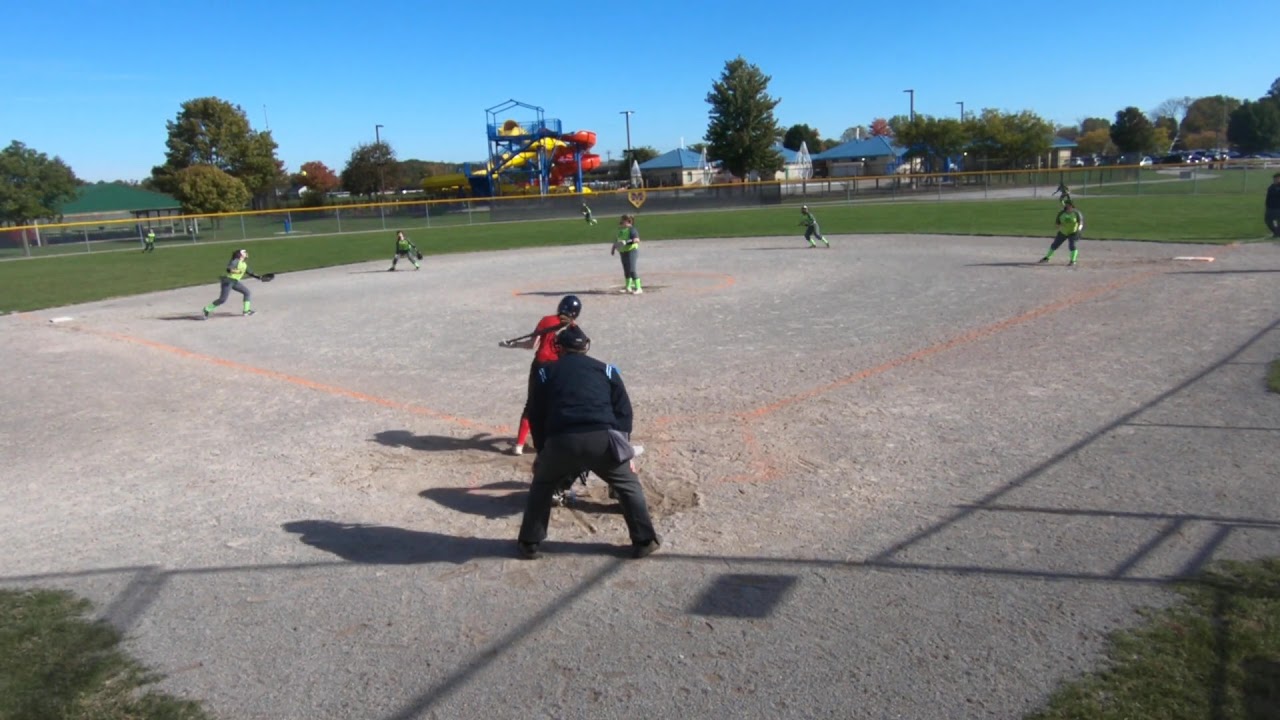The image depicts a lively softball game played on a gray infield with distinctive red base paths. Center stage is the batter in a white uniform who has just completed a swing, closely monitored by an umpire in a dark uniform stationed behind home plate. Although the catcher is obscured by the umpire, a runner or possibly the second baseman, identifiable by a gray and yellow uniform, is sprinting between first and second base. Another official, likely an umpire, is partially visible on the top right in a black uniform. The backdrop features a distant, vibrant playground with a prominent slide, a large tree to the right, and possibly a clubhouse or home nestled behind the center field fence. The sunny weather, marked by a clear blue sky, contributes to the cheerful atmosphere of this engaging scene.